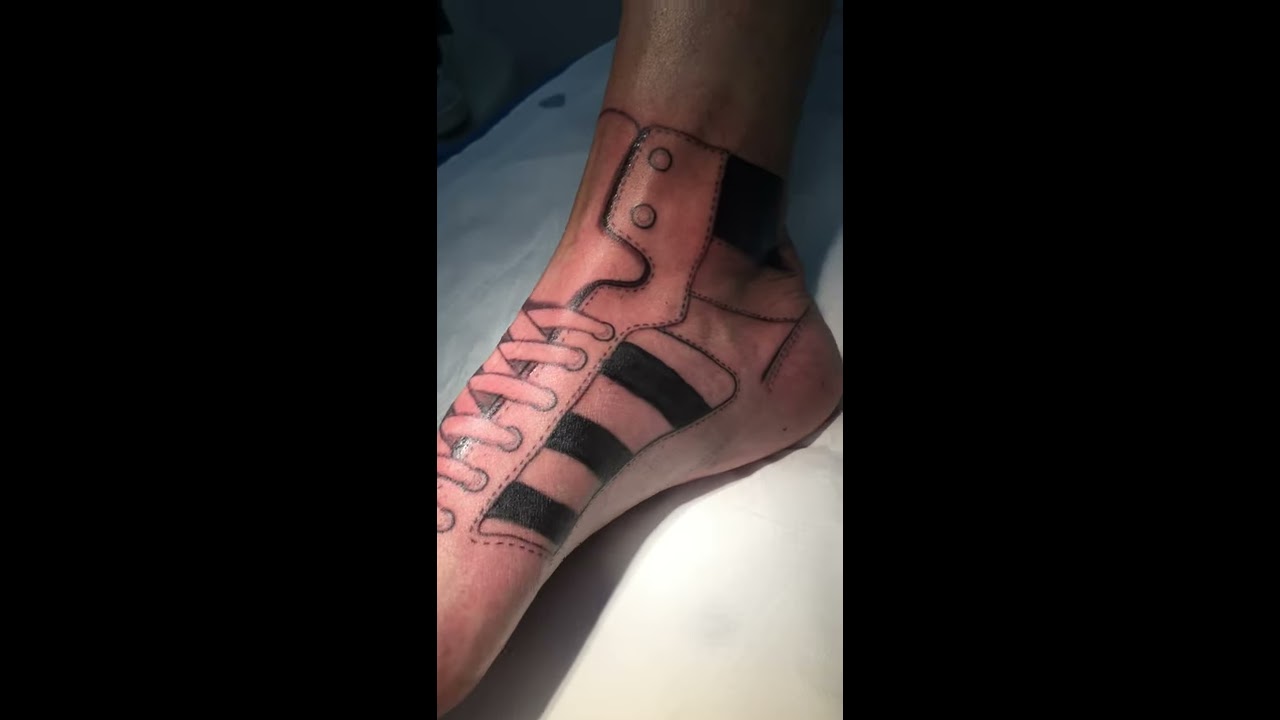The image shows a tattooed right foot placed on a white background, bordered by black rectangles on either side. The tattoo depicts the foot wearing a detailed gym shoe. The tattoo features laces crisscrossed up the center and intricate stitching that outlines the shoe's structure. Near the arc of the foot, there is a logo, and additionally, there are three distinctive stripes along the side. The tattoo also includes a curved spot with two buttons and a dark strip around the ankle. The detailed black ink of the tattoo contrasts with the slightly reddish hue of the leg, suggesting that the tattoo might be freshly done.